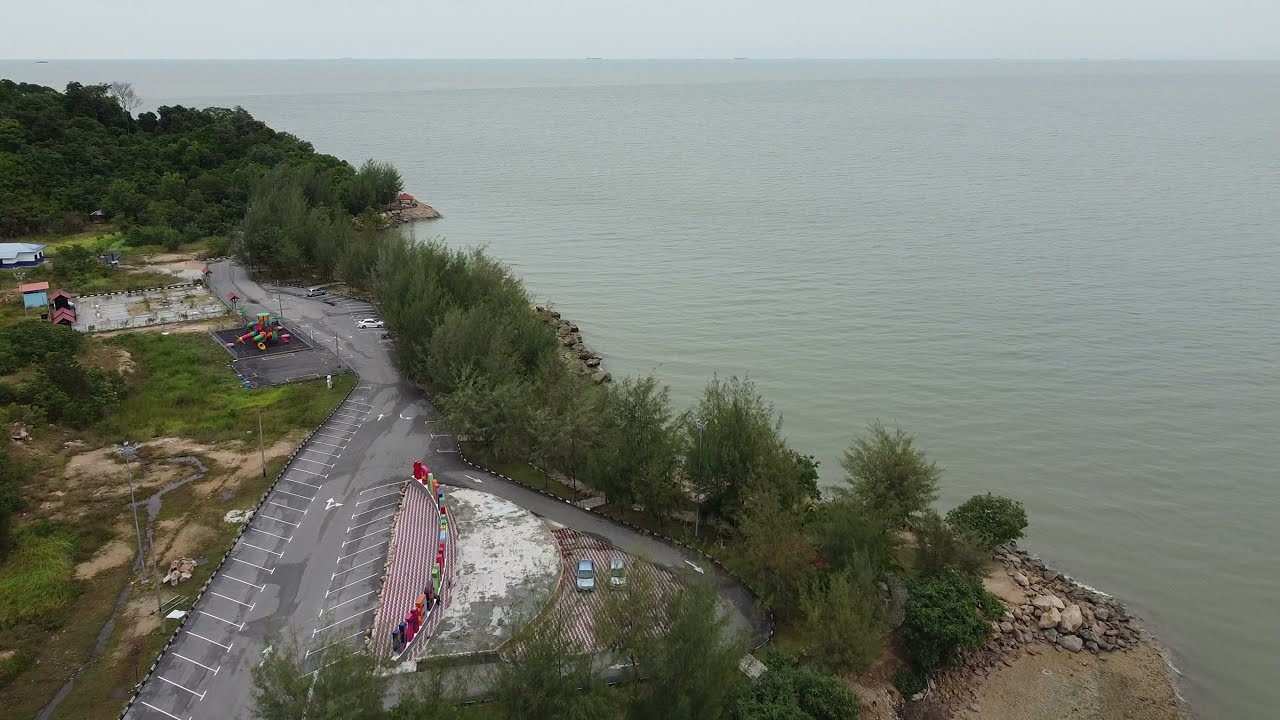This aerial photograph captures a serene shoreline, likely of a large lake or calm ocean, defined by its distinct grayish-blue waters. The shoreline is rocky with a lush line of green trees that abruptly edge a prominent cliff. To the right of the image, the expansive body of water extends, slightly rippled under a hazy blue sky. 

In the foreground, a large, gray parking lot with clearly marked white parking lines is visible, harboring a few cars. A path with directional arrows cuts through the lot, leading down toward the green shrubs bordering the water. Adjacent to this path, a cluster of colorful objects—perhaps playground equipment or facilities—dot the landscape, adding bright splashes of pink, green, and red. 

Behind the parking lot, a road runs parallel to the shoreline, offering access to undisturbed grassy areas and additional trees. Further along, a larger parking area is surrounded by small buildings painted in various hues, including turquoise, orange, and red, standing out against the verdant backdrop. 

Overall, the image illustrates a blend of natural beauty and developed recreational space, meticulously detailing the intersecting elements of water, land, and human infrastructure.